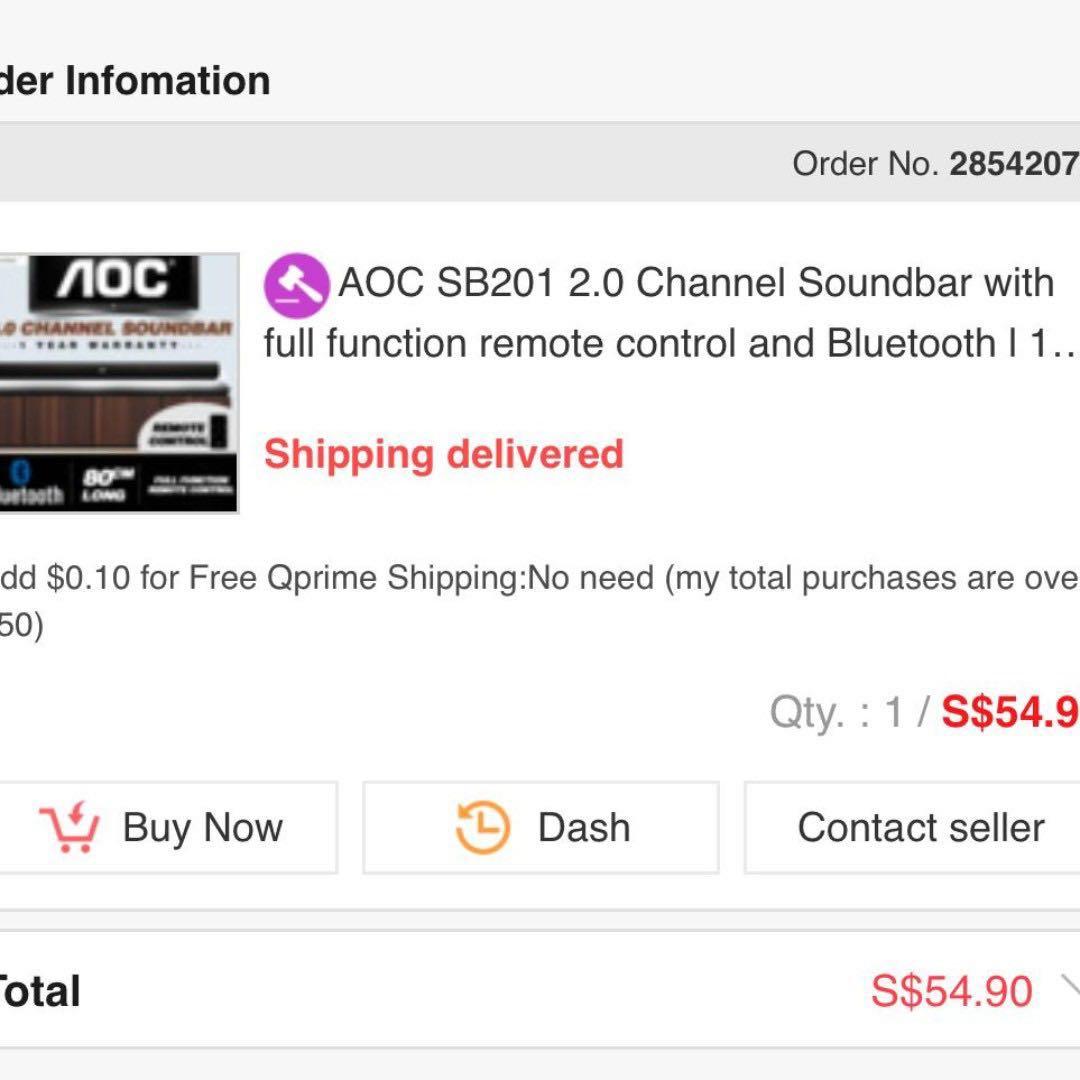The image appears to be a partial screenshot from what seems to be an online retail site, with Amazon being the likely source based on the layout. The focal point of the screenshot is the AOC soundbar, displayed along with its functionalities and a fully functional remote control. However, only half of this product image is visible in the screenshot. The price for the product, including shipping, is prominently listed at $94.90.

The screenshot features several user interface elements typical of online shopping platforms, including a "Buy Now" button and a "Contact Seller" button for addressing any potential issues with the product. The background of the web page is primarily white, enhancing readability and conforming to standard e-commerce design aesthetics. The text indicates the status of "Shipping Delivered," suggesting that the product has already been shipped or is ready for immediate dispatch.